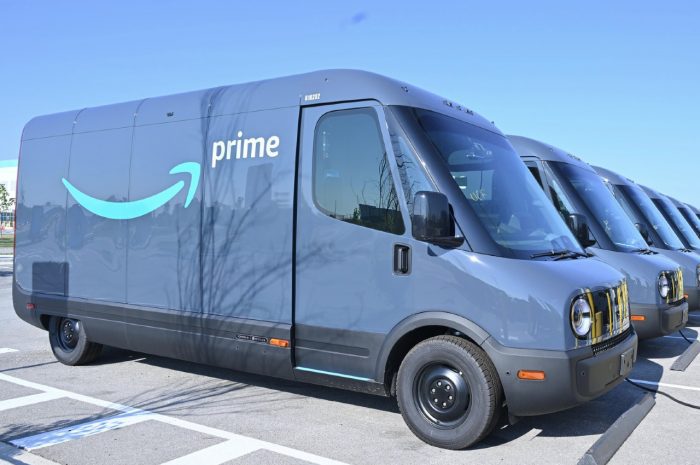This outdoor photograph captures a well-organized scene in a parking lot under a pale blue sky, marred only by a dark wisp of cloud at the center which could possibly be a mark on the lens. In the foreground, the smooth gray asphalt is marked with crisp white lines delineating parking spaces. Dominating the scene are five Amazon delivery vans parked in a precise row, all facing to the right. The focus is on the van at the front, which reveals a striking purple paint job adorned with the recognizable Amazon Prime logo—a white and blue arrow accompanied by the word "Prime" in white text. The partial hoods of the subsequent vans are also visible, maintaining the uniformity and sense of meticulous arrangement.